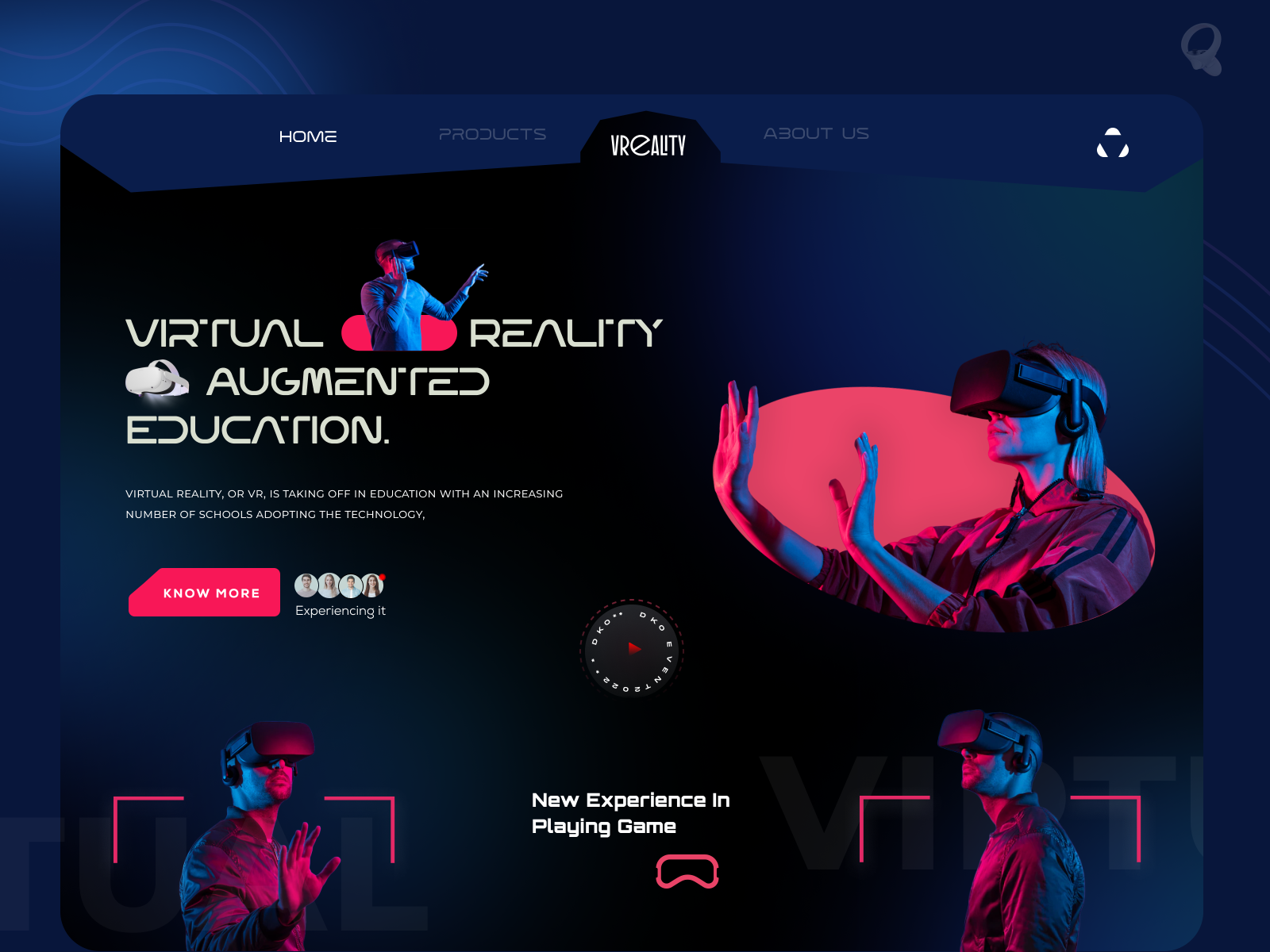On this visually engaging website, the background features a navy blue canvas with gradient shadings — particularly in the upper left-hand corner, where a lighter blue hue suggests a subtle light source. The main interface gives a "website within a website" impression due to its rounded corners.

At the top navigation bar, you'll find options like "Home," "Products," "Virality," and "About Us." The "Virality" section, seemingly a blend of "virtual" and "reality," is currently selected. Below this menu, the content showcases a man with his arms outstretched, wearing a virtual reality headset. Clad in blue, he is likely illustrating the immersive experience of VR. Text accompanying this image reads: “Virtual Reality, Augmented Education,” emphasizing VR's growing adoption in educational settings. Another call-to-action button says "Learn More."

To the right, an image features a young woman engaged in a similar VR experience, her hands outstretched as she interacts with the virtual environment. The caption here states: “New Experience in Playing Games,” indicating VR's extensive application in gaming. The website effectively communicates that while VR is becoming increasingly significant in education, its primary focus remains on gaming experiences.